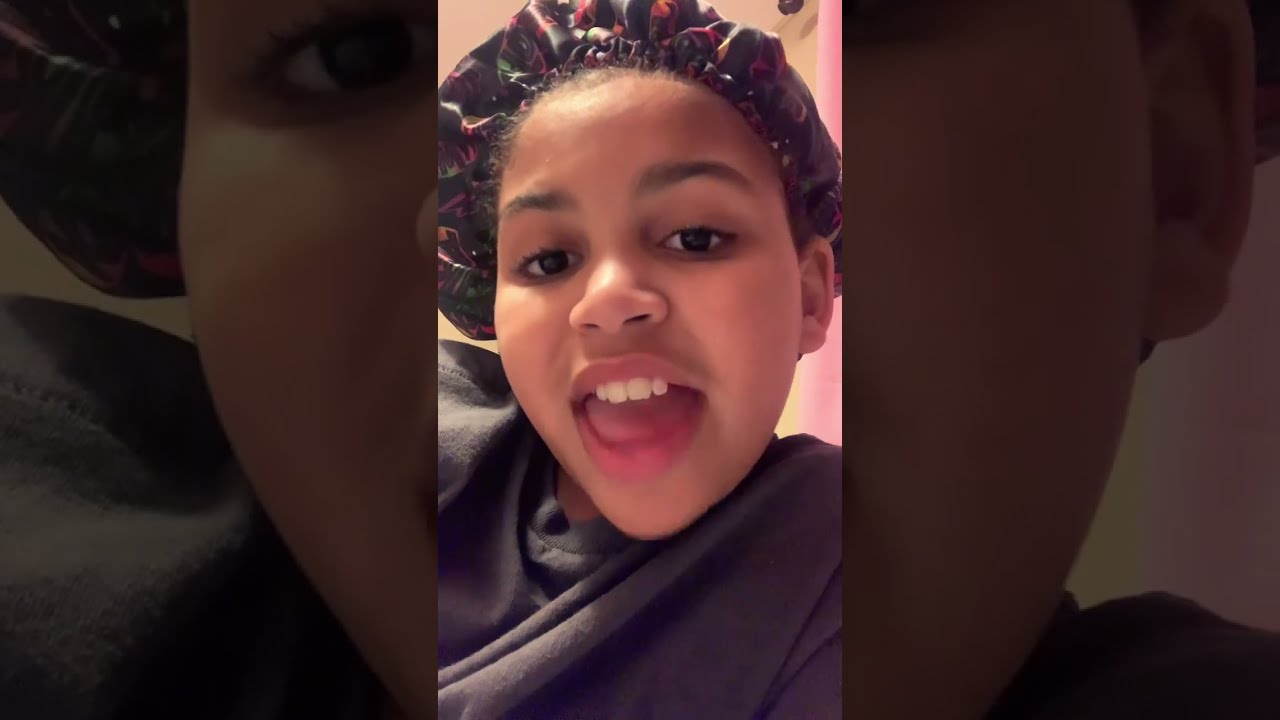This is a highly detailed photograph composed of three panels. The left and right panels are translucent close-ups of the central image, which is backlit and highlighted. Dominating the center of the composition is a young African-American girl with a vibrant, happy expression. Her mouth is slightly open, revealing the top row of her teeth, while her tongue partially obscures the bottom portion of her mouth. She wears a dark silk bonnet adorned with intricate red and purple patterns, with a few strands of her hair peeking out. Her attire consists of a black t-shirt or pullover, which may appear like a robe in some interpretations. The background features a subtle peach or pink-colored wall with light poking through. The central image is of higher quality and not as darkened as the surrounding panels, creating a striking contrast. The entire photograph measures about 9 inches wide by 5 inches tall.